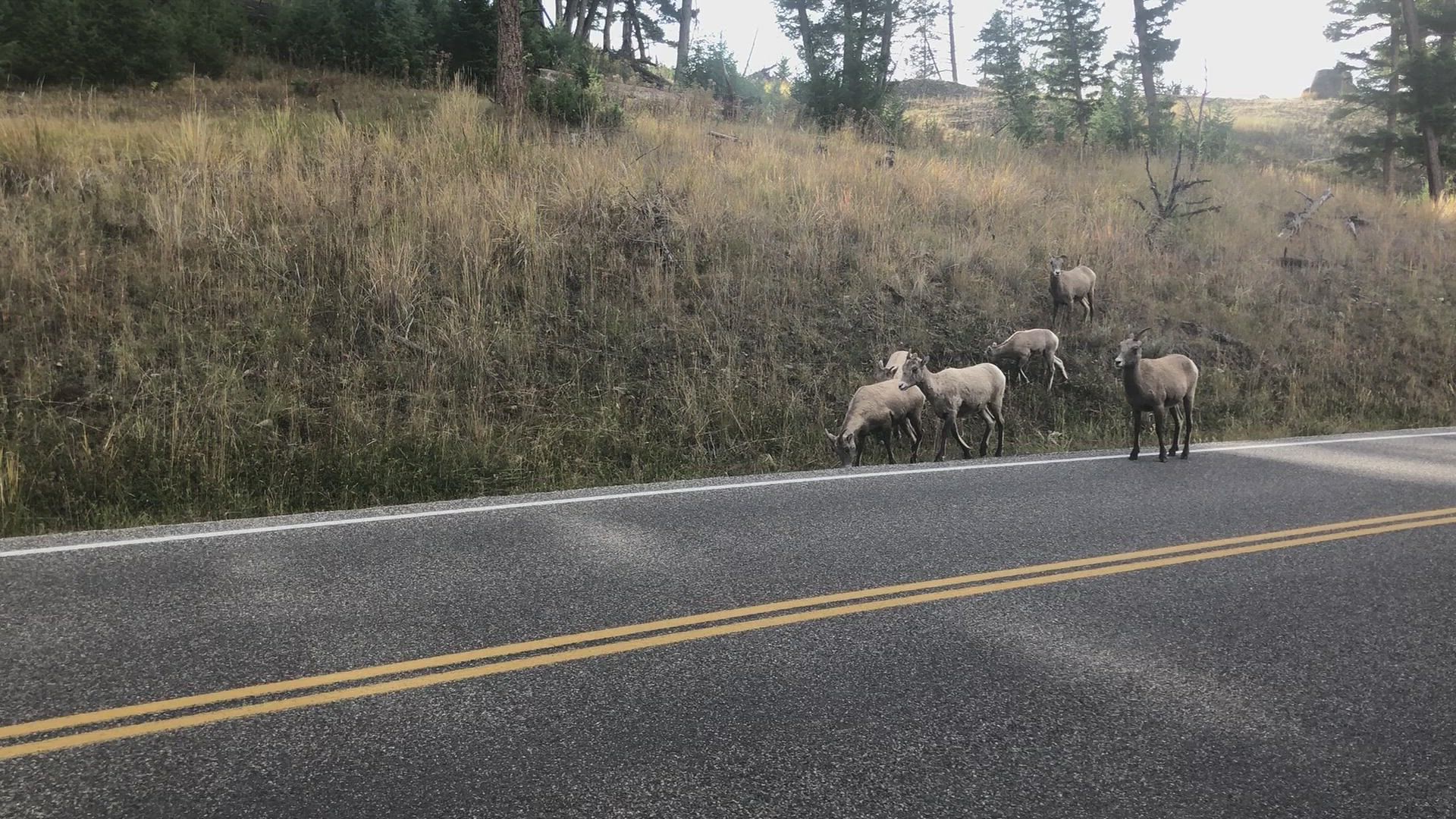A serene scene depicts an asphalt road stretching from the left to the right in the foreground of the image, delineated by dual yellow lines at its center and a white line marking the edge. On the far left side, five light brown goats graze peacefully on a grass-covered hill, interspersed with shrubs. The background reveals a lush landscape of more hills adorned with green shrubs and stately trees, under a clear, expansive sky.